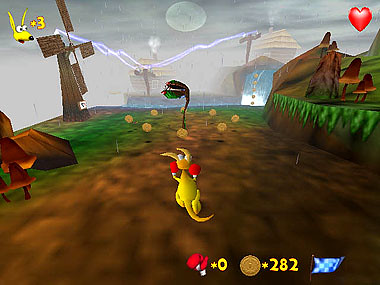A vibrant screenshot captures an immersive moment in a 3D platformer game reminiscent of classic titles like "Jak and Daxter." The central focus is on the main character, a yellow kangaroo donning red boxing gloves, viewed from behind as it stands on the rain-soaked ground. The kangaroo's tail is slightly curved, adding to the dynamic feel of the scene. Surrounding a grey, otherworldly plant, a series of glowing rings float, enhancing the mystical ambience of the game’s world.

To the left of the screen, an inset HUD element displays a portrait of the kangaroo’s head accompanied by the number "3," possibly indicating lives or a similar metric. On the right side of the screen, another HUD element features a heart icon, likely representing the character's health. Below this, a series of numbers and symbols provide additional gameplay information, though their exact function remains unclear. The overall rain-slick environment, vivid character design, and detailed interface elements combine to evoke a rich, nostalgic gaming experience.